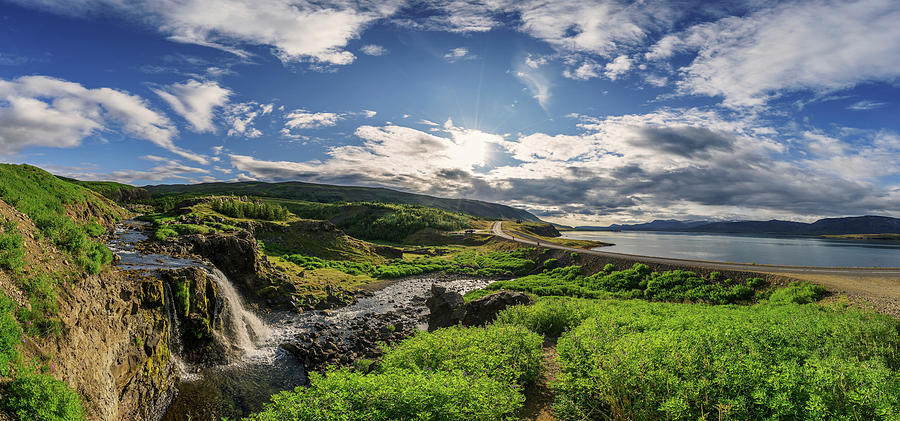The panoramic landscape shot captures a vibrant, untouched wilderness under a bright blue sky dotted with large, fluffy clouds that partially shield the sun, casting a soft light over the scene. Dominating the right-hand side is a wide, winding river, its distant shore just barely visible, adding a sense of depth and vastness. Adjacent to the river is an unpaved road that cuts through the landscape slightly right of center, flanked by a grassy, uneven foreground marked with patches of brown and mud. To the left of the road, a rocky terrain covered with brush slopes upward to a rocky elevation, from which a stream cascades down in a picturesque waterfall. In the distance, a row of blue-green mountains or highlands rise behind the river, creating a sublime backdrop that encapsulates the serene beauty of this natural setting.